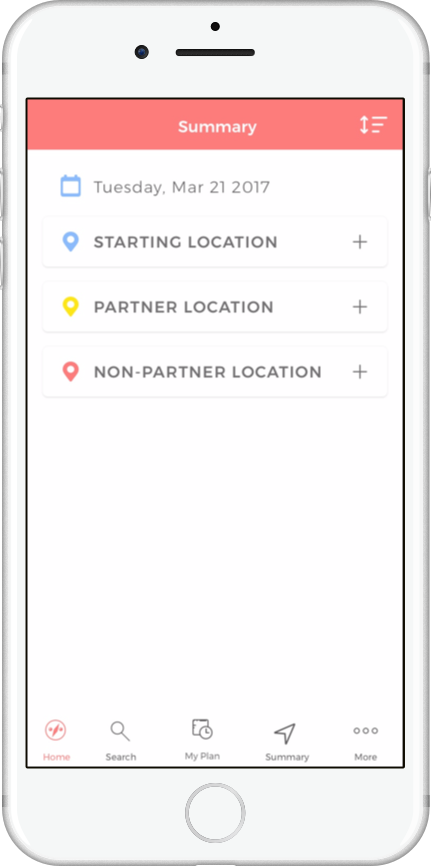The image depicts a screenshot of a white iPhone, likely an older model given its thin and flat design. The iPhone's screen displays an app interface with a predominantly white background. At the top of the screen, there's a red-bordered header labeled "Summary," followed by the date "Tuesday, March 21, 2017." Below this header, there are three listed items with distinctive colored icons: a blue checkpoint labeled "Starting Location" with a plus sign, a yellow icon labeled "Partner Location," and a red icon labeled "Non-Partner Location."

Toward the bottom of the screen, a navigation bar features five options: "Home," "Search," "My Plan," "Summary," and "More." This interface appears digitally enhanced as opposed to being part of a natural background, indicating that the elements were edited into the image.